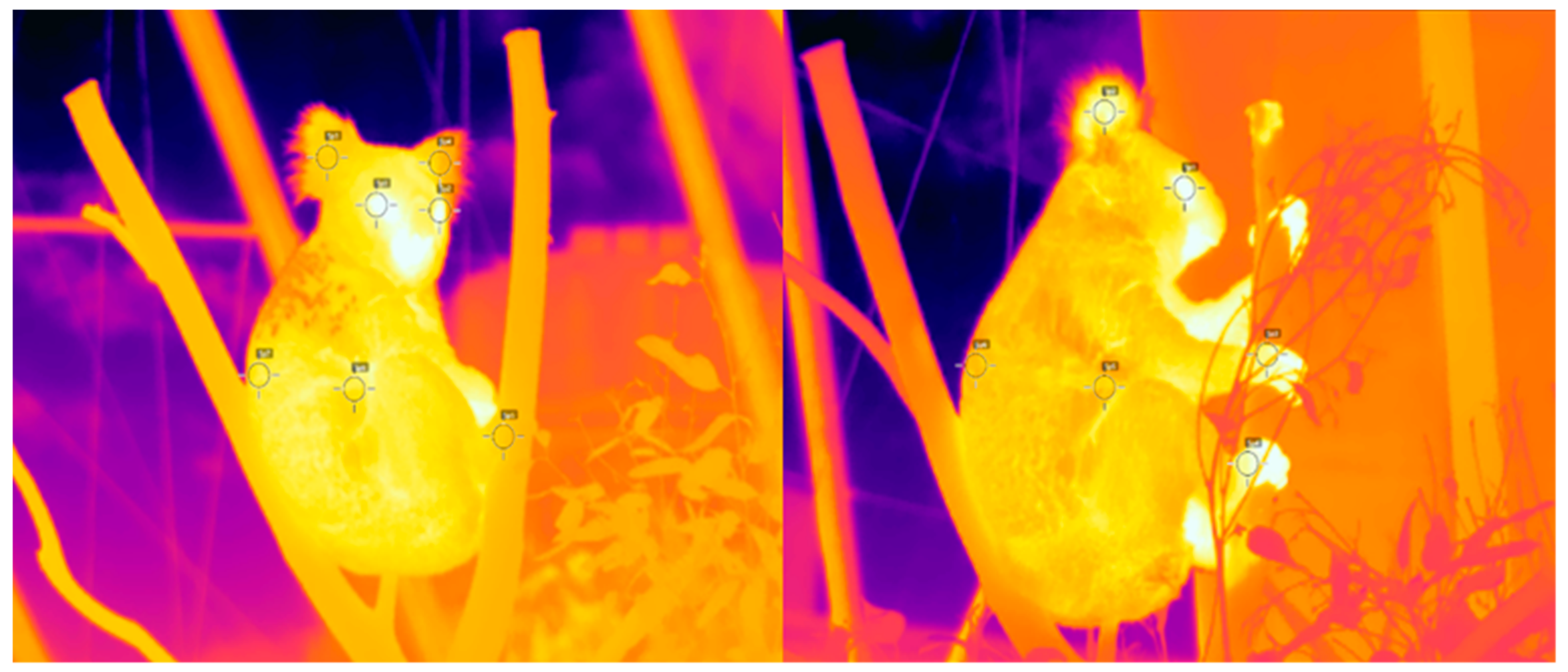The image comprises two side-by-side thermal photos of a koala positioned in a tree, depicted in vibrant thermal imaging colors. The koala, identifiable by its characteristic shape and behavior, is shown holding onto branches, which appear orange and yellow in the thermal spectrum. In both photos, the animal has white highlights on its face, paws, and other warmer body parts, accentuating the heat distribution. The background of the images transitions from deep purples and blues, indicating cooler areas, to oranges reflecting warmer objects like the leaves and branches.

In the left photo, the koala faces the camera, giving a clear view of its white-highlighted eyes and mouth, while in the right, it turns to focus on the tree. The overall color palette includes bright pinks, neon yellows, oranges, reds, and whites against a colder purplish-red backdrop, with some areas marked by target signs likely indicating temperature readings at specific points, such as the ears, joints, and eyes. These distinct thermal visuals emphasize the warmness of the koala's body against the cooler night environment captured in the photos.